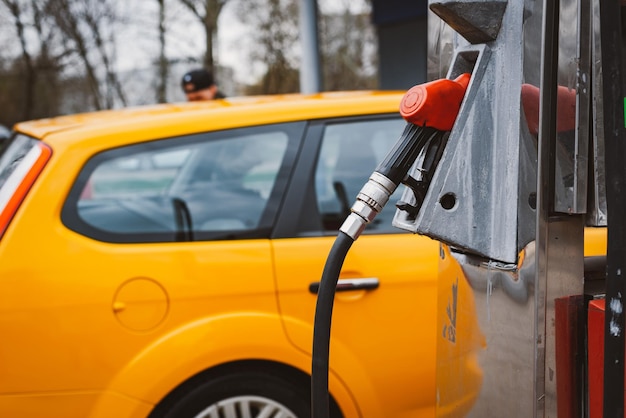This full-color photograph, taken outdoors on an overcast day, captures a scene at a gas station. Dominating the image is a vintage yellow station wagon, possibly from the 1970s or 1980s, positioned at a gas pump on the right side of the frame. The station wagon, facing right, showcases its rear quarter panel and back door with a clear, large glass hatchback window. The black right rear tire is partially visible along with the gas cap indentation. 

Adjacent to the car, the tall, steel-gray metal gas pump features a secured black hose with a red nozzle resting in its holder. Surrounding this main scene, bare trees with some leaves are visible, set against a muted gray sky. Through the car's windows, a person standing beside the vehicle is seen, their head slightly left of center, wearing a dark hat or beret. The photograph is devoid of borders, enhancing its natural, staged, and detailed composition.